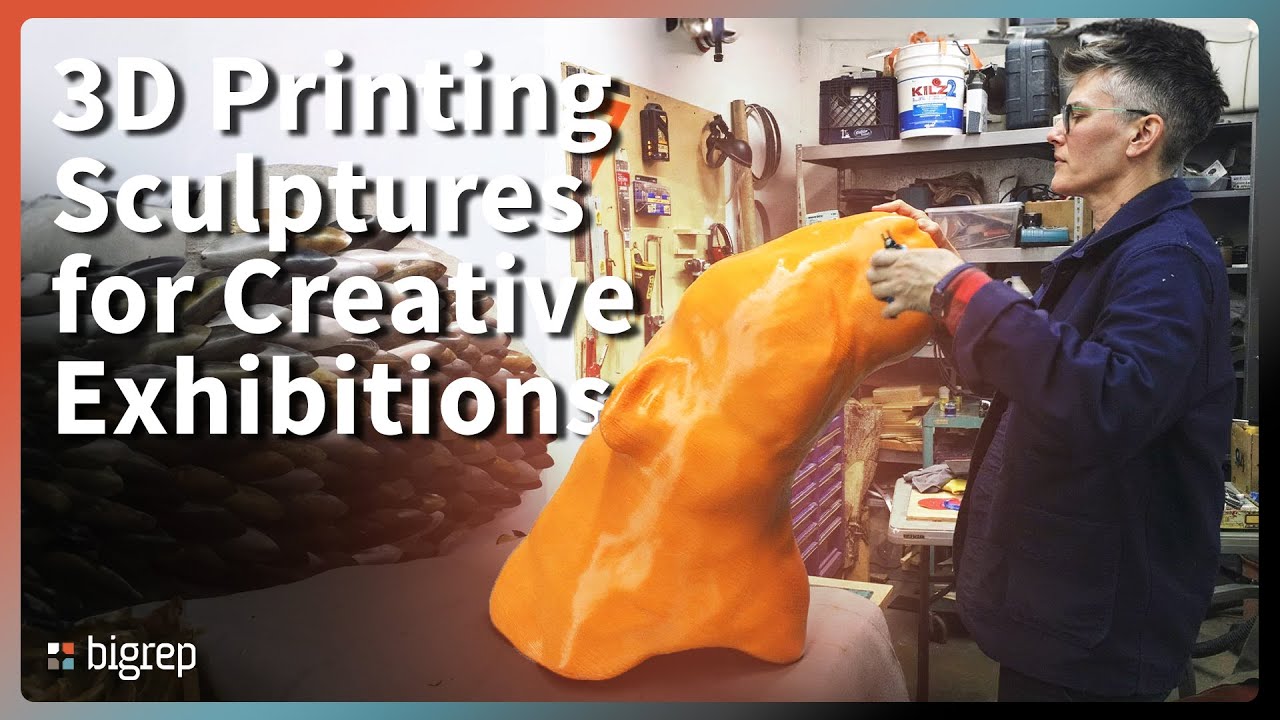In this image, we see a detailed scene inside a workspace captured within a horizontal rectangular frame. Dominating the center is a woman in her early 40s with a very short black and white pixie cut. She is focused on molding a large, orange structure roughly as tall as her waist—a cylindrical shape bending over to the right. The woman, clad in a blue jacket, is holding a sculpting utensil in her left hand while her right hand rests atop the mold.

White letters prominently read "3D Printing Sculptures for Creative Exhibitions" along the left side of the image, with "Big Rep" in white text positioned in the bottom left corner beside four colored squares. Behind her, shelves are visible holding containers, plastic bins, and an assortment of sculpting supplies. Additionally, various tools hang neatly on the wall. Adding to the visual interest, the image is bordered with red on the left and blue on the right sides.